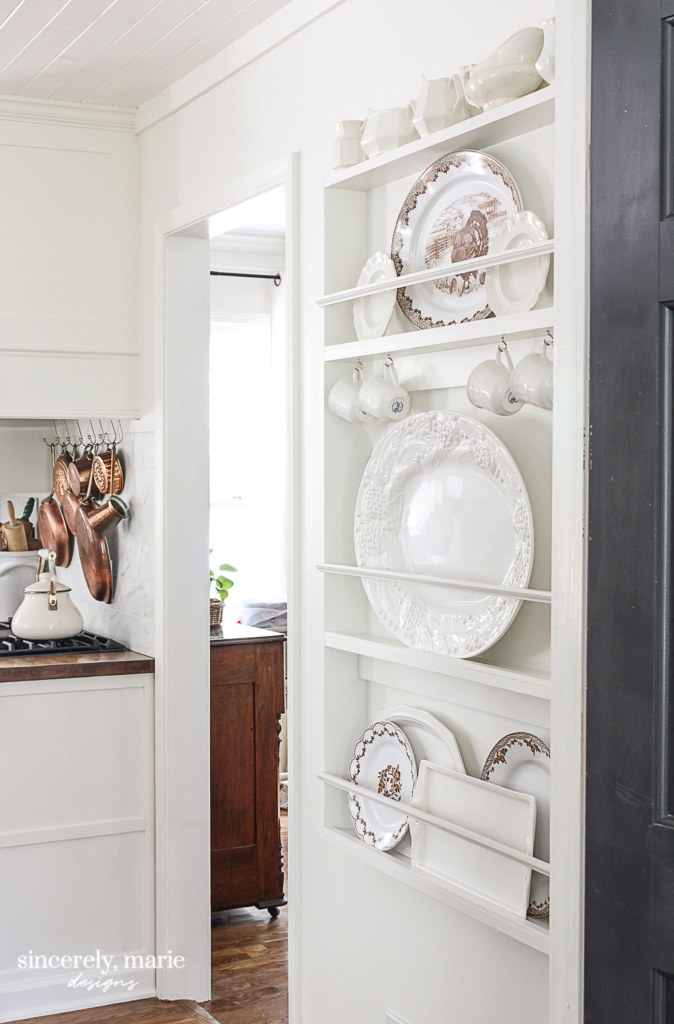The image depicts a quaint, farmhouse-style kitchen with a sliding barn door, accentuating a blend of rustic and vintage design elements. The barn door, positioned on the left side of the photo, is open, revealing a room beyond that features a wooden credenza adorned with a green plant and partially-obscured sunlight streaming through a window with a black curtain rod. The door itself showcases built-in shelving with neatly arranged kitchenware: the top shelf holds creamer bowls, sugar and creamer bowls, while the second shelf displays three plates, including a central plate adorned with a turkey design. Below, there is a larger alcove with four coffee cups flanking a beautifully designed large white platter. The bottom recess holds a rectangular platter accompanied by four circular platters, all secured by a bar.

Within the kitchen, the atmosphere is bright and airy, characterized by white walls and a sense of clean organization. The counter features a white teapot with golden handles, adjacent to three small and two larger copper pans hanging on the wall. A white porcelain utensil basket containing a rolling pin sits behind the teapot. Additionally, built-in shelves display vintage plates and scalloped serving trays, with smaller trays and teacups hanging below. The lower left-hand corner of the photo is marked with the signature "Sincerely Marie Designs." The overall decor exudes a medieval, coquette vibe with a farmhouse charm, highlighted by the presence of copper cookware against a marble backsplash.